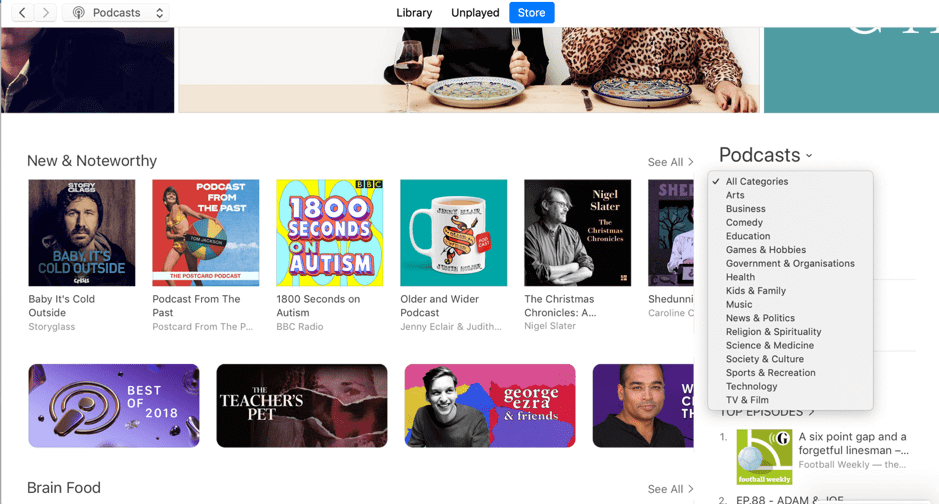This image displays a laptop screen open to the iTunes application, specifically the Podcasts section. In the top left corner, the word "Podcasts" is prominently featured. At the top center of the screen are three tabs: "Library," "Unplayed," and "Store," providing easy navigation options for the user. Beneath the "Podcasts" header, a comprehensive list of categories is shown, including:

- All Categories
- Arts
- Business
- Comedy
- Education
- Games and Hobbies
- Government and Organizations
- Health
- Kids and Family
- Music
- News and Politics
- Religion and Spirituality
- Science and Medicine
- Society and Culture
- Sports and Recreation
- Technology
- TV and Film

Each category offers a wide range of podcast genres to suit various interests, allowing the user to explore and select their preferred content easily. The overall layout is user-friendly, making podcast discovery and organization straightforward.